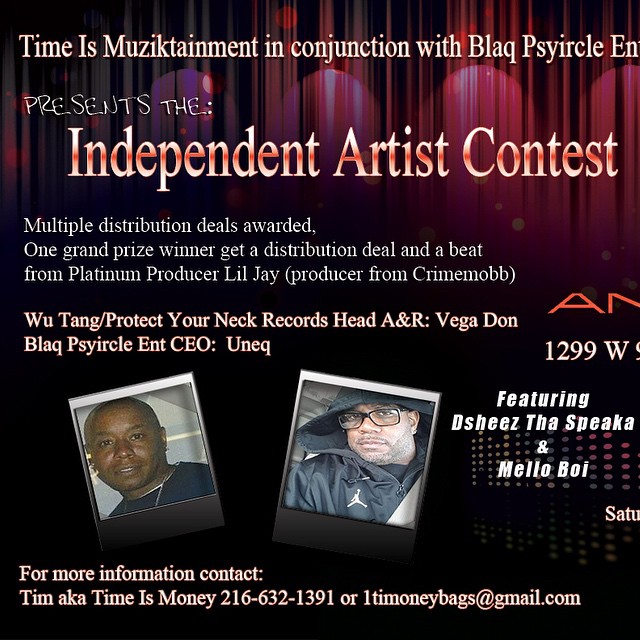The image is a detailed poster announcing the "Independent Artist Contest," presented by "Time is Music Tainment" in conjunction with "Black Circle EN." The background features a stage with drawn curtains in shades of pink and red, and stage lighting is visible on the sides. The text at the top reads "Time is Music Tainment in conjunction with Black Circle EN," followed by "Presents the Independent Artist Contest" in bold, brightly colored fonts on the backdrop.

The headline states, "Multiple Distribution Deals Awarded," and announces that one grand prize winner will receive a distribution deal and a beat from platinum producer Lil Jay, known from Crime Mob. Further details include mentions of "Wu Tang/Protect Your Neck Records head A&R Vega Don Black Circle and CEO UNEQ."

Below this, two Polaroid-style images are displayed: one of a black man in a blue t-shirt and the other of a person in a black hoodie with glasses and a trimmed beard, seemingly seated in a car with a seatbelt on. The sides of the image feature partial texts which include names "Deshiz the Speaker" and "Mellow Boy," presumably the people in the pictures.

At the bottom of the poster, a contact information section is provided: "For more information contact Tim aka Time is Money" along with a phone number, "216-632-1391," and an email address, "timemoneybags@gmail.com." Various text elements are presented in multiple font sizes, styles, and shapes.